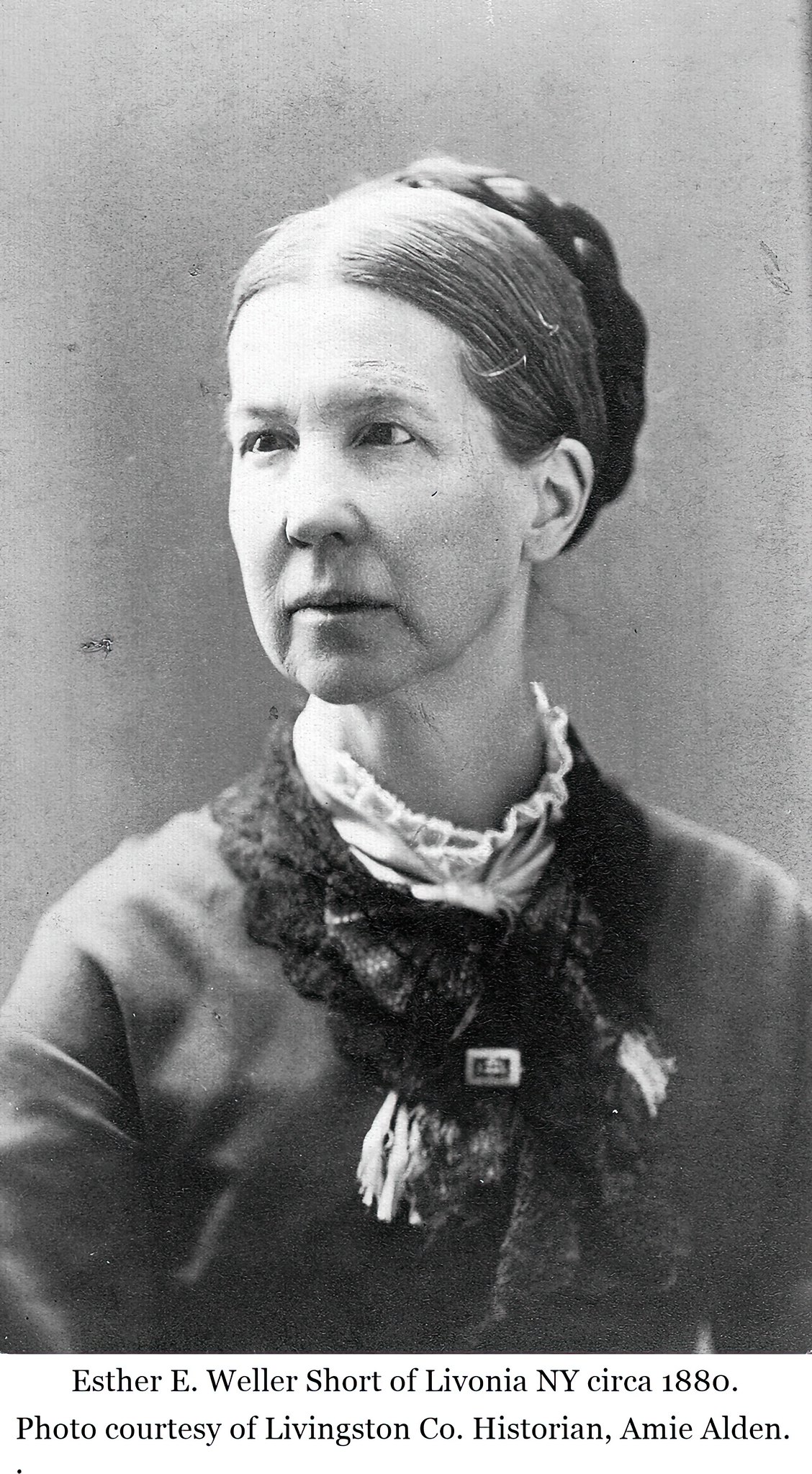This black and white portrait, set against a gray background, depicts a woman from circa 1880. Her light complexion and dark hair, slicked back into a braid wrapping around the back of her head, stand out clearly. Her attire includes a high-collared white shirt beneath a dark, plain dress, complemented by a lace black scarf tied around her neck. The woman gazes to her left, her expression neutral and distant. The image, well-preserved and brightened by natural light, is notably clear. At the bottom, the text reads: “Esther E. Weller Short of Livonia, New York, circa 1880. Photo courtesy of Livingston Co. Historian Amy Alden.”